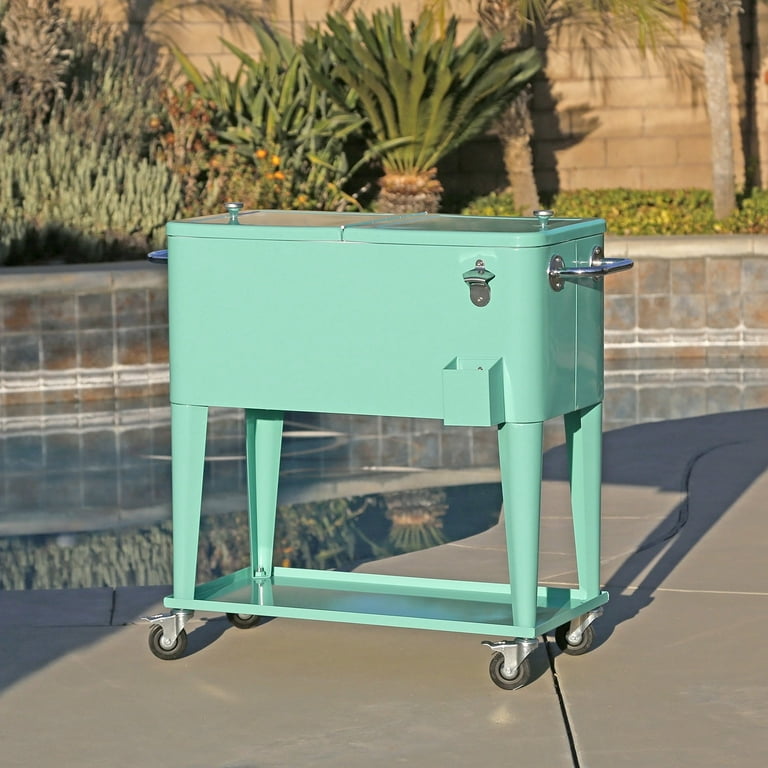In this bright, sunny outdoor scene, a vintage-style rolling cart, painted an aqua reminiscent of the 1950s, stands prominently beside a pool on a grey cement ground. The cart features a rectangular box shape with a silver handle on the right side and stands on four aqua-colored necks, each with a wheel at the bottom. There is an additional tray positioned at the lower part of the cart. The pool's edge is lined with brown tiles, and its walls are made of stone or bricks, creating a rustic look. Across the pool, a brown brick wall with brown mortar serves as a backdrop, adorned with green plants and small yellow flowers. In front of these walls, two pine trees can be seen along with some lower-growing greenery. The cart, which resembles an old cooler or ice cream freezer, hints at summer gatherings and refreshing treats.